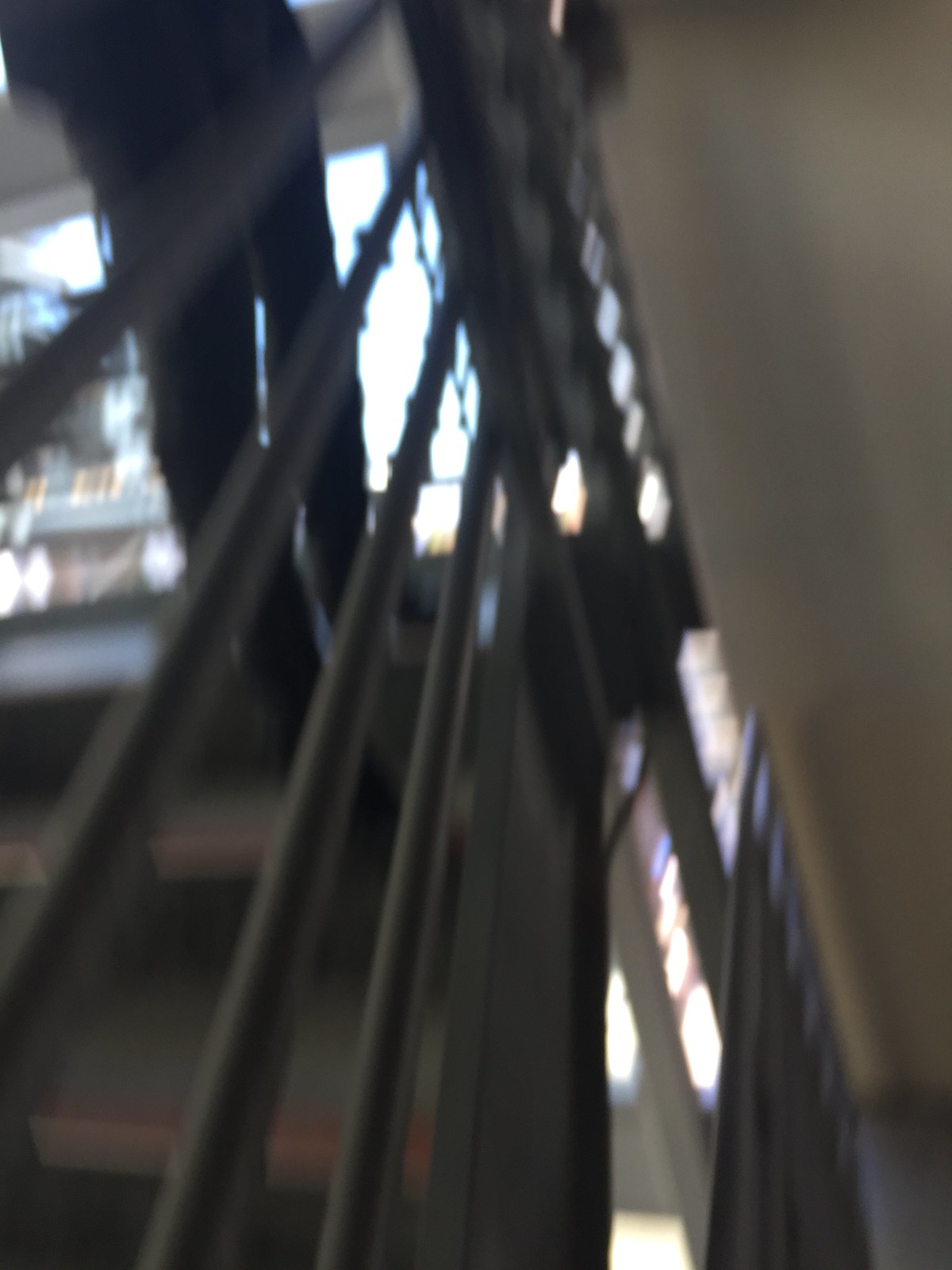In this blurred photograph, the focal point appears to be a stairwell. On the right side of the image, the white ceiling slopes downward, while to the left, metal stairs ascend, featuring four handrails. In the background, large picture windows flood the scene with bright natural light. At the top of the stairs, a figure can be vaguely seen, appearing to be wearing jeans, though the image's blurriness makes details indistinct. The metal stairway seems to be of a considerable width, and there is a shadowy area beneath the stairs where the person might be standing, contributing to the overall contrast in lighting.